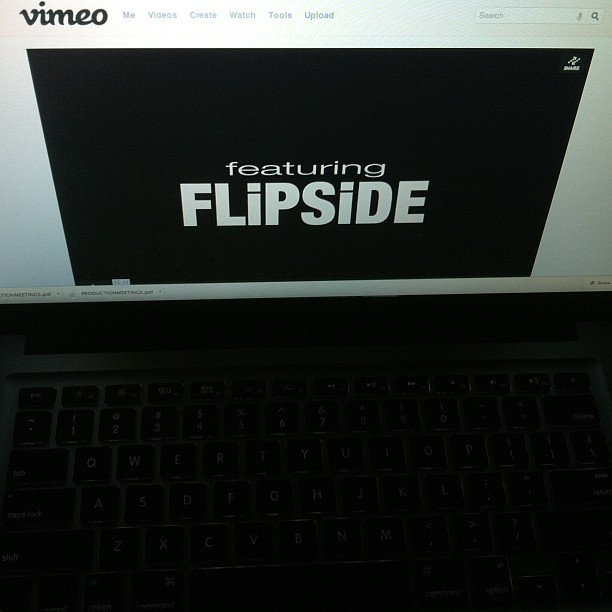The image is a detailed photograph of a laptop screen displaying the Vimeo website. The screen shows a video titled "Featuring Flipside" in white text on a black background. The Vimeo menu is visible at the top of the screen, with options for Me, Videos, Create, Watch, Tools, and Upload, along with a search bar in the top right corner. The Vimeo logo can be seen in the upper left. The laptop keyboard is visible but partially obscured by darkness, revealing barely discernible keys with white lettering. The computer seems to be running a Windows operating system, as suggested by the visible taskbar at the bottom of the screen. Overall, the photograph captures a moment of paused activity on the Vimeo website.